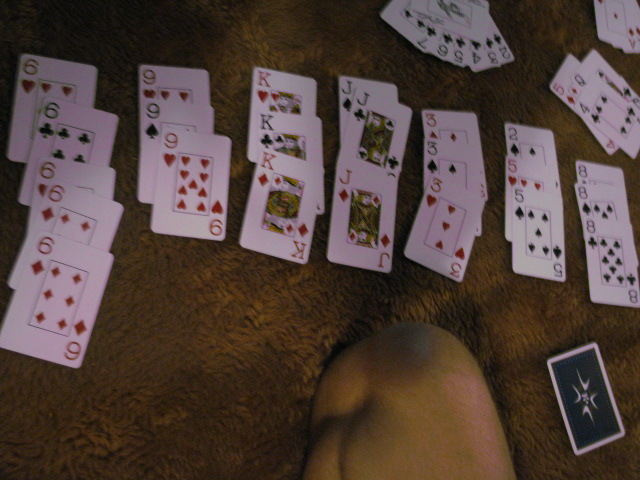This photograph captures a somewhat cluttered scene centered on a person crouching on a black carpet. Only the person's leg is visible, specifically a bent knee, suggesting they are kneeling. The individual's knee, which appears noticeably large, hints that the person may be slightly overweight, with some flabs around the knee area.

The primary focus, however, is on the playing cards meticulously spread out on the ground. The cards extend from the left to the right and are also present in the top right corner of the frame. On the far left, one card displays multiple sixes. Next to it is another card adorned with several nines, followed by a card with numerous K's. Continuing from left to right, the sequence features cards with three J's, three 3's, a 3 and a 5 together, another 5, a 3 and a 6 combination, and finally an 8.

In the top right section, a collection of cards is fanned out, though they are all upside down. This area also contains small stacks of cards: one stack consists of three cards, and another has two cards. Additionally, there is a card face down at the bottom right of the image. While this card doesn’t appear to be a typical playing card, it features a black back decorated with several arrows pointing towards its center.

The precise arrangement of the cards and their varied formations suggest they may be part of a strategic layout or a game in progress, though the exact significance of the numbers and groupings remains unclear.